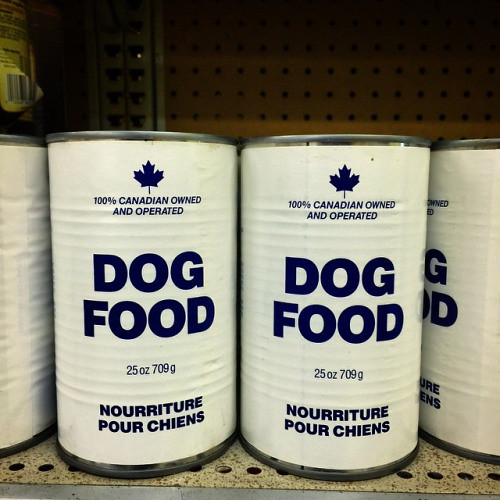The image captures a close-up of a store shelf, prominently displaying cans of dog food. At the center of the shelf are two cans, with additional cans of the same brand extending to both the left and right. Each can features a plain cream-colored label. At the top center of the label, there is a Canadian maple leaf emblem. Below this emblem, the text reads "100% Canadian owned and operated," followed by a larger font stating "Dog Food." In smaller font beneath this, the weight is indicated as "25 ounces (709 grams)." At the bottom of the label, the phrase "Nourriture pour chiens" is printed, translating to "nutrition for dogs" in French. The metal shelf has a series of perforations, and the background displays a pegboard commonly used for hanging shelf hooks.